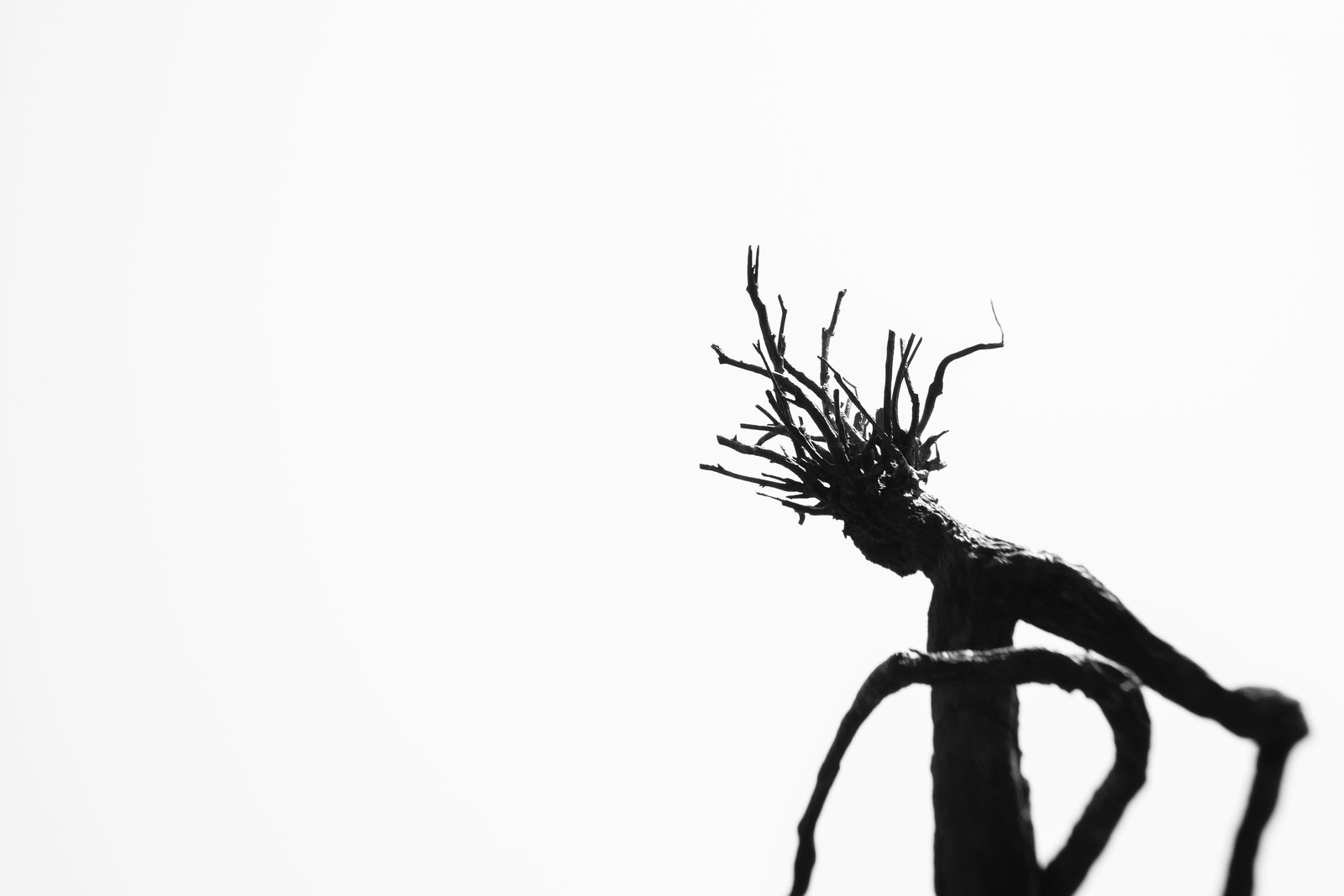The wide rectangular image depicts a black, metal-like sculpture resembling a human figure, positioned in the bottom right corner against a faint off-white background. The sculpture captures the upper body of a person with a torso extending from the bottom of the frame and an arm reaching diagonally downwards. The head is tilted down towards the bottom left, adorned with several spiky, branch-like extensions that curl at the ends, giving the appearance of a crown. The texture of the sculpture is reminiscent of tree bark, and it reflects light, adding to its intricate details. A curved object encircles the torso, starting from the bottom and extending behind. The convergence of human and natural elements in the form of branches and bark-like texture adds depth and intrigue to the statue, making it a captivating focal point.